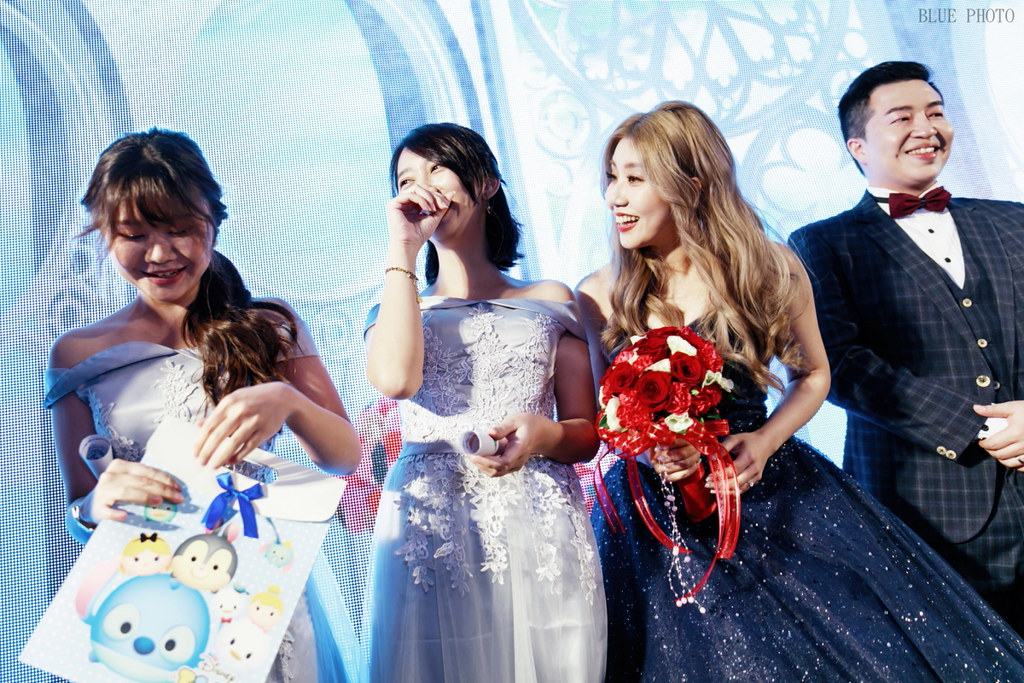In this vibrant and celebratory image, four people are standing on a stage with a mesmerizing LED backdrop showcasing a winter-inspired palace scene, reminiscent of a Frozen setting. From left to right, the first woman is dressed in a strapless lilac gown adorned with floral patterns, holding a large envelope embellished with a ribbon and Disney character cartoons. She has brown hair and appears to be looking down at her card. The second woman, laughing and cupping her right hand towards her mouth, is in a strapless dress nearly identical to the first, but with white floral designs. She has black hair and wears a black bracelet. Next to her, the third woman stands out in a sparkling dark blue strapless gown decorated with silver sequins, holding a bouquet composed of mainly red and white roses, her blonde hair adding to her radiant appearance as she laughs joyfully. Finally, on the far right, is the sole man in the picture. He dons a checked dark blue suit paired with a red bow tie and has black hair. Unlike the women, he looks off to the right, away from the camera, adding a touch of intrigue to the scene. All four seem to be sharing a moment of happiness and laughter, beautifully capturing the spirit of the occasion.